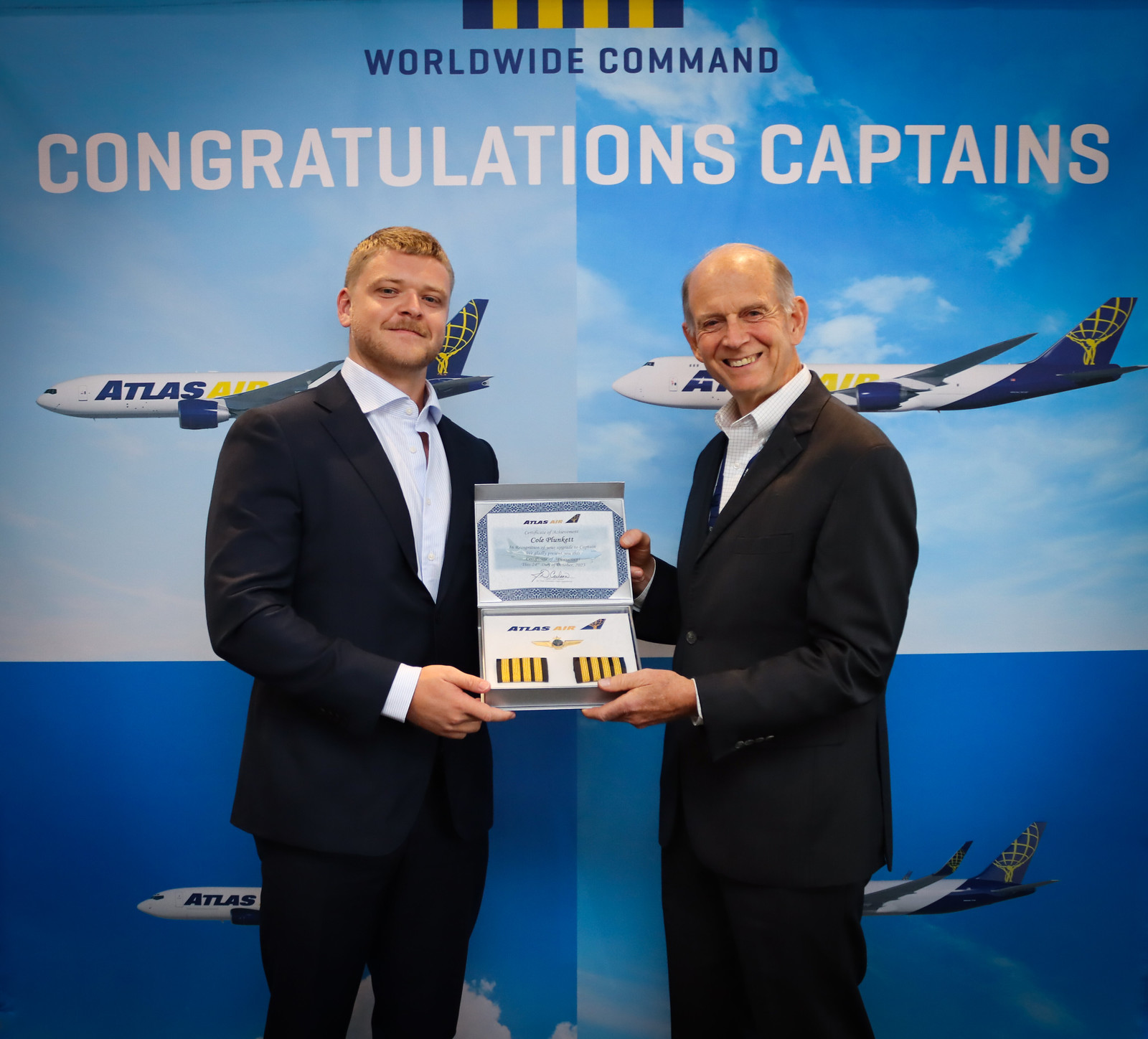The photograph features two men standing before a large, detailed poster. The poster is split into four squares, each depicting a sky with an airplane flying through it. The top part of the poster is light blue while the bottom part transitions to a darker, electric blue. Each airplane bears the Atlas Air logo, with "Atlas" in blue and "Air" in yellow. Above the images, a small rectangle with blue and yellow stripes is visible, accompanied by the text "Worldwide Command" in blue and "Congratulations Captains" in white.

The man on the left is younger, with short blond hair and a blond mustache. He is dressed in a navy blazer, a light-colored collared shirt, and black pants. He is smiling directly at the camera while holding an award or certificate in his right hand.

The man on the right, older and balding with some gray hair on the sides, is wearing a gray or black suit and a white collared shirt. He is also smiling, revealing his teeth, and is positioned so that his body is turned slightly to the left while his head faces forward. He holds the award or certificate with his right hand at the top and his left hand at the bottom. Both men are posing proudly in front of the poster.